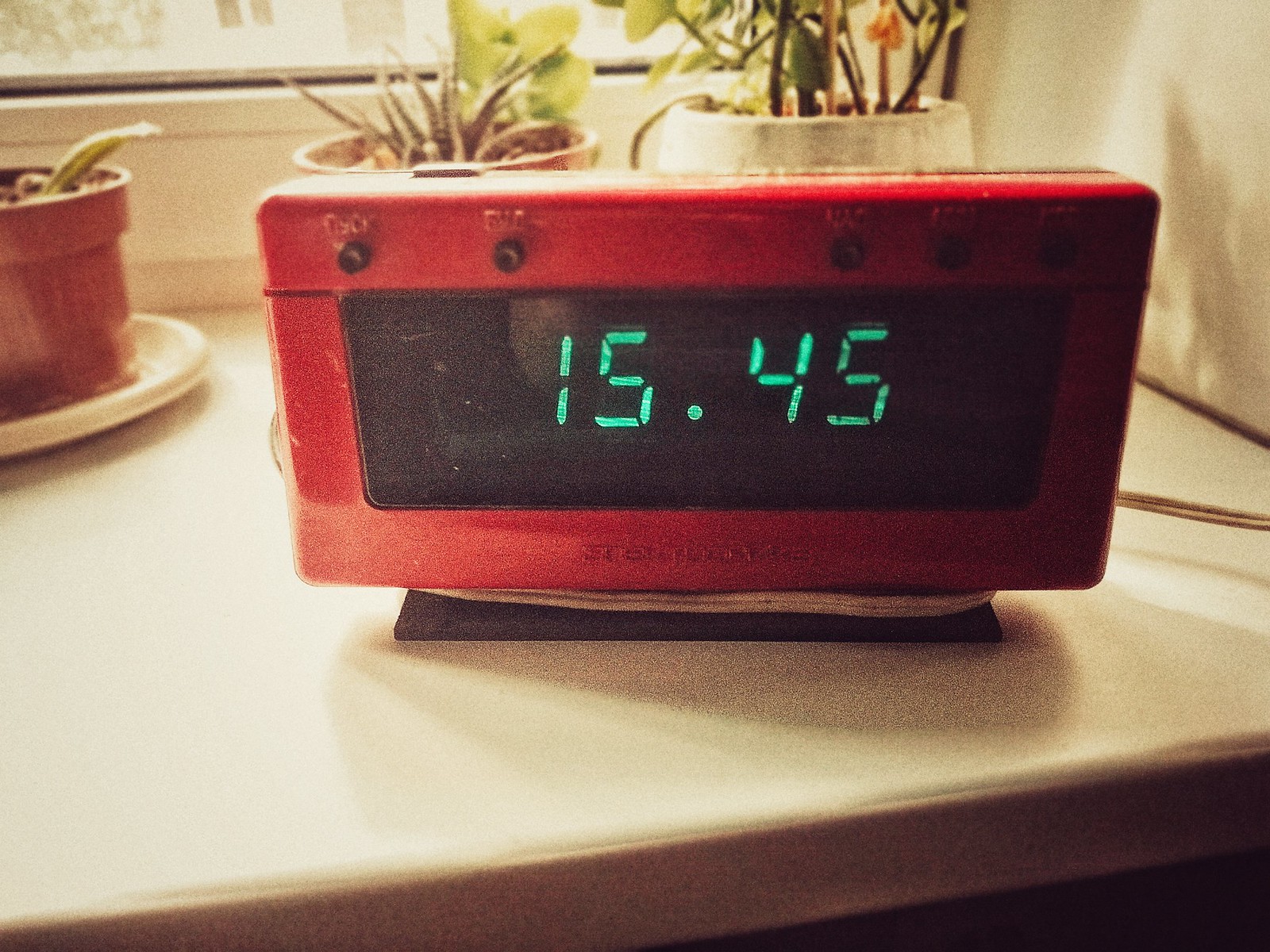This color photograph captures a close-up of a digital clock, its tones appearing somewhat desaturated, likely due to a filter or artificial lighting. The clock, rectangular in shape with a red outline, features various knobs: two on the left and three shadowed knobs on the right. Small, unreadable lettering is located at the center bottom of the clock. The focal point is a large black screen displaying the digital time "15:45" in vibrant green numbers. The clock is supported by a metallic and black stand, positioned on a whitish shelf. A cord extends from the right-hand side of the clock. The background includes two potted plants: one in a whitish pot directly behind the clock on the right, and another in a brownish pot. Additionally, part of another pot plant in a brownish pot with a white saucer is visible towards the left-hand corner. Above, the bottom of a white window completes the scene.